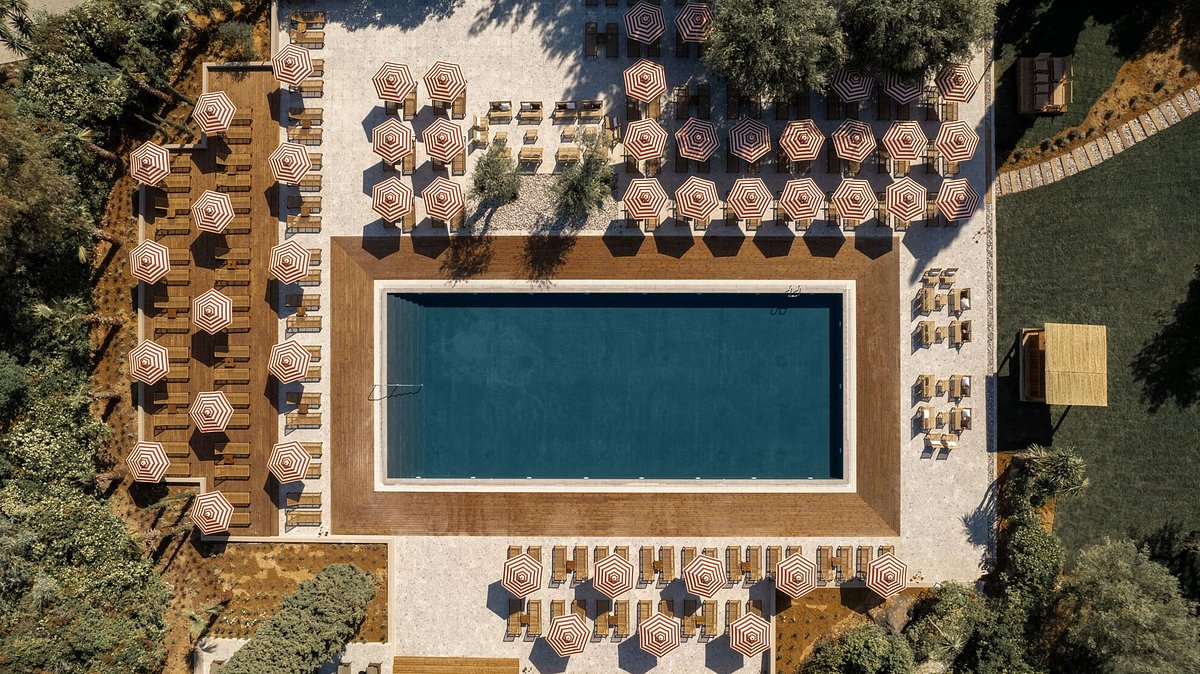This aerial view, likely captured by a drone, showcases a large, rectangular swimming pool with a distinctive golden border around its white concrete edges. The serene pool scene is situated in what appears to be a resort setting, surrounded by numerous umbrellas and beach chairs perfect for sunbathing. On the left side of the pool, a cluster of tables with umbrellas provides a shaded retreat, similar to the arrangement found at the pool's far end. The right side also features lounge chairs under umbrellas, with an additional small cabana structure visible. Trees dot the landscape, bordering the scene, and a broad road can be seen on the right, likely leading back to the main resort or hotel area. The image captures a bright, sunny day, reflected in the sharp shadows suggesting it’s around mid-morning. Despite the inviting setting, no one is currently in the pool. A green lawn with trees and a wooden structure can be seen in the broader view to the right.